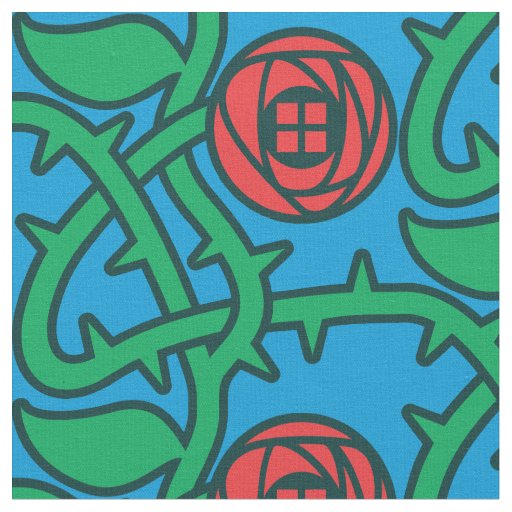The image is an artistic rendition of a rose bush set against a light blue background. The drawing features green, curved stems adorned with green leaves and thorns. At the tips of the stems, there are red, circular roses. The more prominent flower on the right is fully visible, displaying intricate black lines within its petals, and inside the flower, a distinctive black circle contains a simple four-pane window-like design formed by red squares. To the left, partially visible, is another rose, sharing the same vibrant red and black detailing. The composition is enclosed within a square frame, giving it a structured yet organic feel, reminiscent of a tattoo-style design.